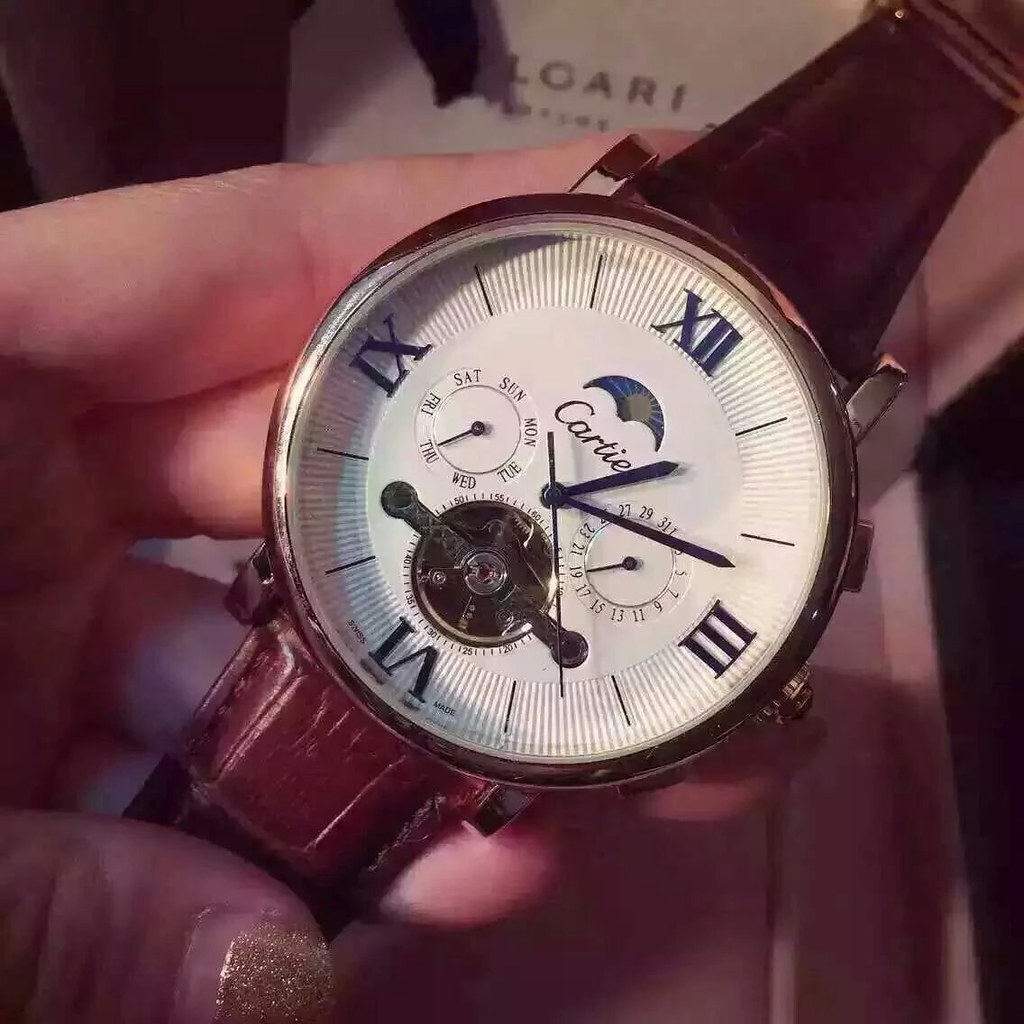This image showcases an up-close, detailed view of a wristwatch held by a Caucasian hand adorned with sparkly gold nail polish on the thumb. The watch, positioned diagonally from the bottom left to the top right corner of the frame, features a dark brown leather strap attached to a gold casing. The face of the watch is predominantly white, accented with Roman numerals at the 12, 3, 6, and 9 positions, while the other hours are marked with simple dashes. The watch hands are black, with a thicker long hand, a thicker short hand, and a thin long hand indicating the time, which is around 1:17. Additionally, below the 12 o'clock position, the word “Cartier” is inscribed in cursive. The face also seems to display complications for the days of the week and the dates, adding to its sophisticated design. The background of the image reveals a bit of white space at the top, potentially showing partial text or branding.